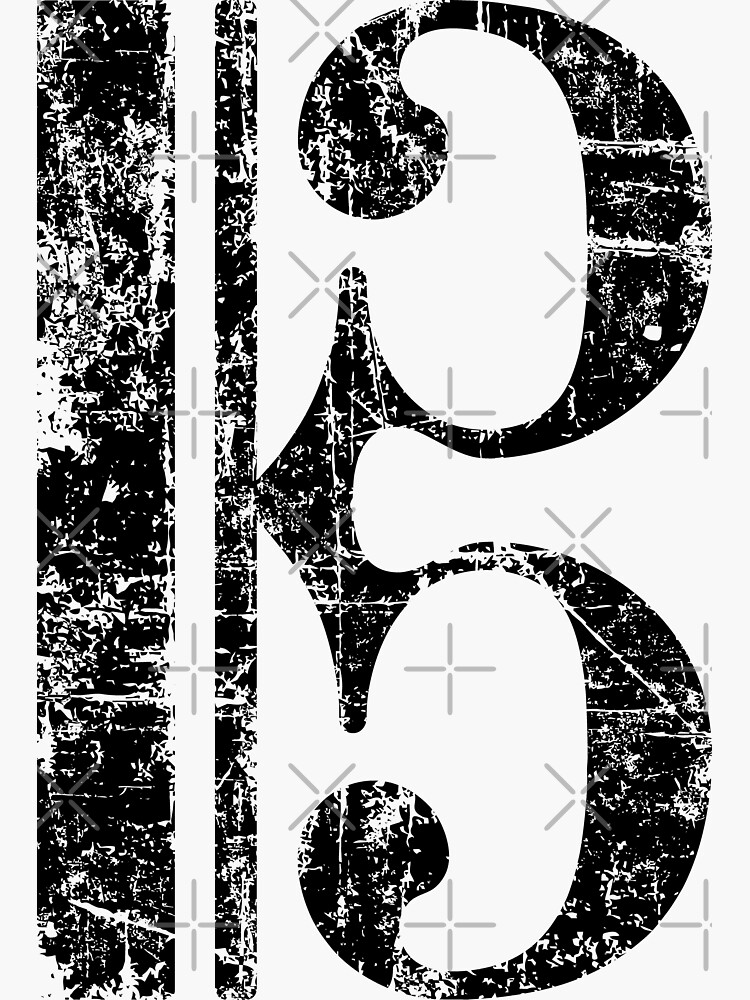In a rectangular, portrait-oriented image that is roughly one and a half times taller than it is wide, a white background is adorned with alternating columns of gray pluses and X's. These gray crosses are arranged such that one column features plus signs while the adjacent column displays the same symbols rotated to form X's, creating a subtle pattern across the background. Over this backdrop, multiple elements of a black, worn-looking design are laid out. Starting from the left, there is a broad black vertical bar marked with random white patches that resemble abrasive markings. Adjacent to this is a thinner white strip dotted with a few gray crosses, followed by another narrow black bar showcasing the same abrasion pattern. Further to the right, and extending to the edge of the image, is a black shape that intriguingly resembles an Art Deco interpretation of the number three. This shape, which could also be likened to a decorative handle or a door knocker, features complementary white abrasion marks and connects centrally to the thinner black vertical line. The combination of these abstract elements creates a visually complex and textured composition within the image.